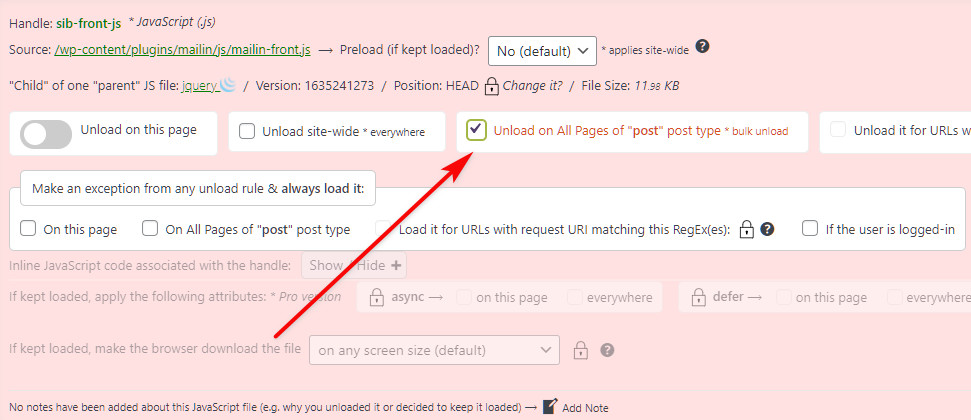**Descriptive Caption:**

The image showcases a configuration screen with an arrow pointing towards a specific field. The field pertains to the bulk unload settings for a JavaScript file named "mail-in-front.js," which is located in the "wp-contents/plugins/mail-in/js" directory. The screen provides an option to preload the file with an unchecked toggle for "kept loaded by default". A note at the bottom indicates that no comments have been added about this JavaScript file, including examples of why it was unloaded or the rationale for keeping it loaded. Options on the screen allow for exceptions to be made to any unload rule, ensuring that the file always loads on specified post types or URLs matching a given regex pattern.